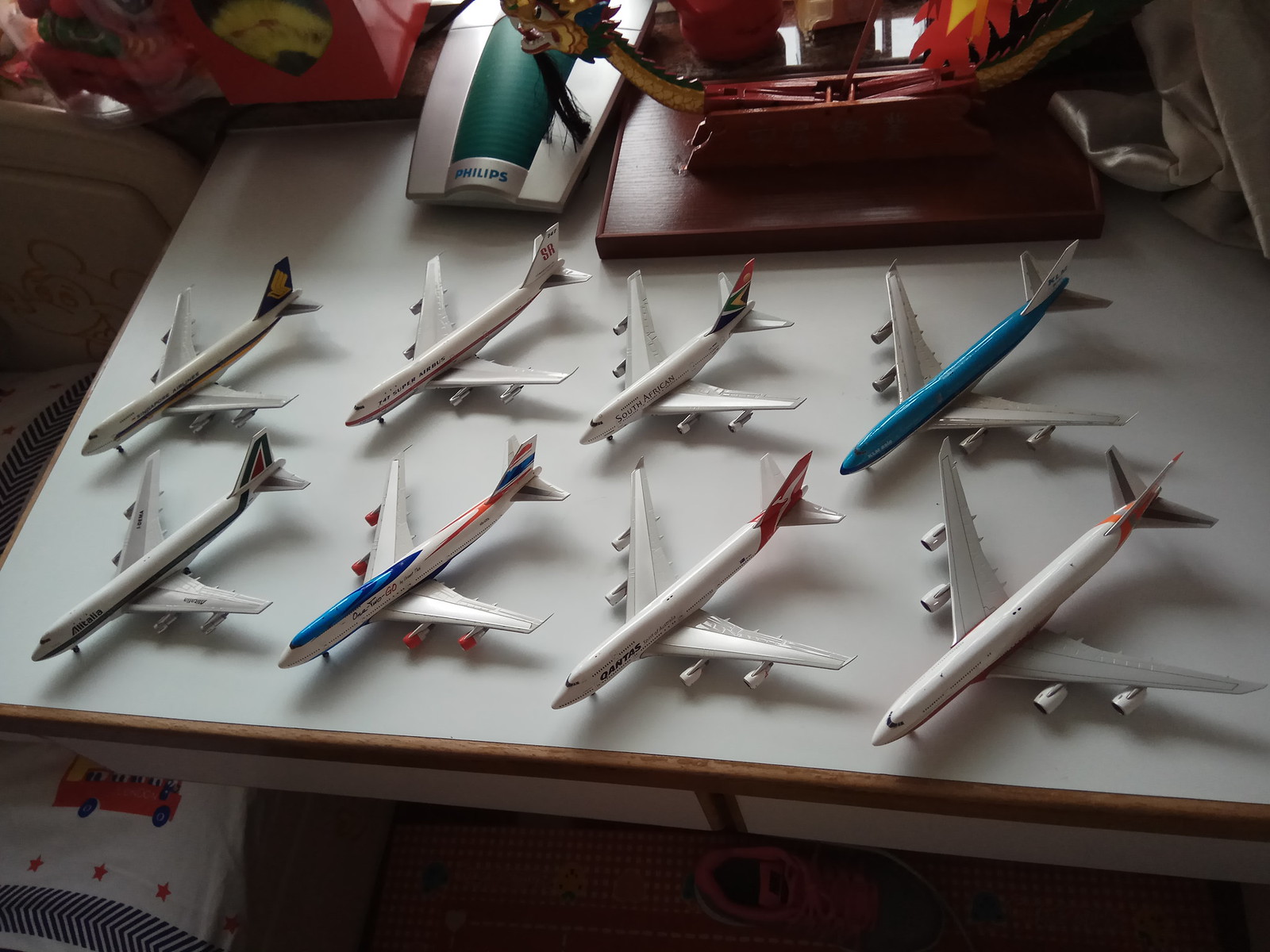The image showcases a white table with a wood grain border set in what appears to be a child's room, next to a bed on the left. Atop the table, there are eight model jet airplanes, each roughly the size of a human hand, arranged to face the bottom left corner of the photo. 

The planes predominantly feature white fuselages with multicolored accents. Notably, two planes stand out with blue bodies and gray-tipped wings, distinct from the other mostly white-and-red models. The planes' tails vary: one has a dark blue tail adorned with gold, another marked "SR" in red, and a third displays the African flag with vibrant hues of black, yellow, green, red, and blue. One of the front-row jets has a blue streak near its cockpit and orange detailing around its jet engines.

Behind the table, a gray and green Philips device, possibly a phone base, is visible along with a wooden decorative object that resembles a dragon's head. Below the table, a blanket with a child-like drawing of a school bus, complete with black wheels, windows, and possibly passengers, adds to the room's playful atmosphere. The blanket also features three red stars and a pattern of alternating blue rectangles and triangles.